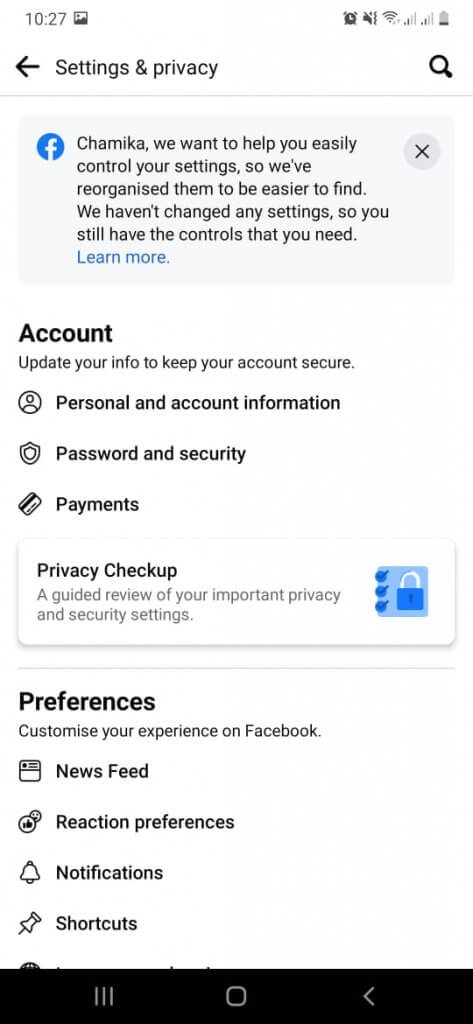This is a detailed screenshot of a user’s phone displaying a section of the Facebook app related to settings and privacy options. At the very top, the phone's status bar displays the time as 10:27, alongside icons for a picture, Wi-Fi, battery life, and data signal strength. 

Directly below the status bar, the header reads "Settings & Privacy" with a search icon on the right side. The main content begins with a blue-framed box featuring the Facebook logo and a message: "Shamika, we want to help you easily control your settings so we've reorganized them to be easier to find. We haven't changed any settings so you still have the controls that you need. Learn more."

Following this, there's another white box with the heading "Account" in bold black text. The content within this box emphasizes the importance of updating personal information to keep the account secure, with sections labeled "Personal and Account Information," "Password and Security," and "Payments," each accompanied by small relevant icons.

Further down, there's another section titled "Privacy Checkup," described as a "guided review of your important privacy and security settings," which is visually supported by a small blue lock icon.

The last section is "Preferences," which offers options to customize the user experience on Facebook. These options include "News Feed," "Reaction Preferences," "Notifications," and "Shortcuts."

At the very bottom of the screenshot is a rectangular black box containing three horizontal lines, a square, and an arrow.